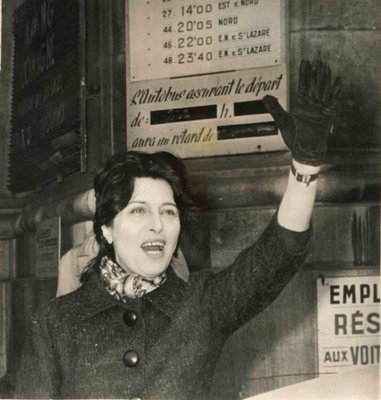This is a vintage black-and-white, slightly sepia-toned photograph likely from the 1950s or 1960s, depicting a solitary woman positioned slightly off-center. Her attire is elegant, featuring a dark, buttoned-up overcoat with large buttons and a hint of a scarf peeking out from above the collar. She sports dark gloves and a watch on her raised left hand. Her short, dark hair appears to be pulled back slightly, and her mouth is open as if she's speaking or calling out. The woman is angling slightly towards the camera, her arm extended upward with her palm forward, suggesting she may be waving or attempting to hail a cab. Behind her stands a wooden wall adorned with signage predominantly in French, indicating that the setting is likely in France. One sign features rows and columns of numbers and partial text, potentially related to bus or train schedules, with visible letters such as 'EMPL', possibly short for 'employee'. She is the sole subject of the image, giving it a timeless and focused narrative.